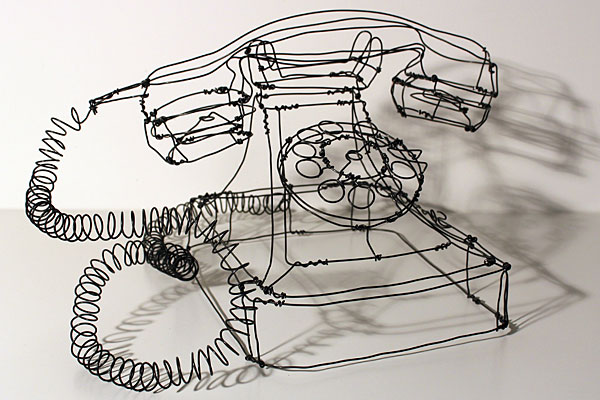This is an image of a 3D sculpture of an old-fashioned rotary telephone made entirely from thin black wire. The wire forms a detailed outline of the classic telephone, including a square base, a raised portion with circular dials, and a receiver that rests on the cradle when not in use. The wire receiver is connected to the base by a coiled wire cord, intricately crafted to resemble the original phone's coiled cable. The entire sculpture is transparent, allowing visibility through its frame, and it casts distinct shadows on the gray wall and the surface it sits on, due to lighting from the left side. The background and the surface on which it rests are grey, highlighting the black wire construction against the neutral backdrop.